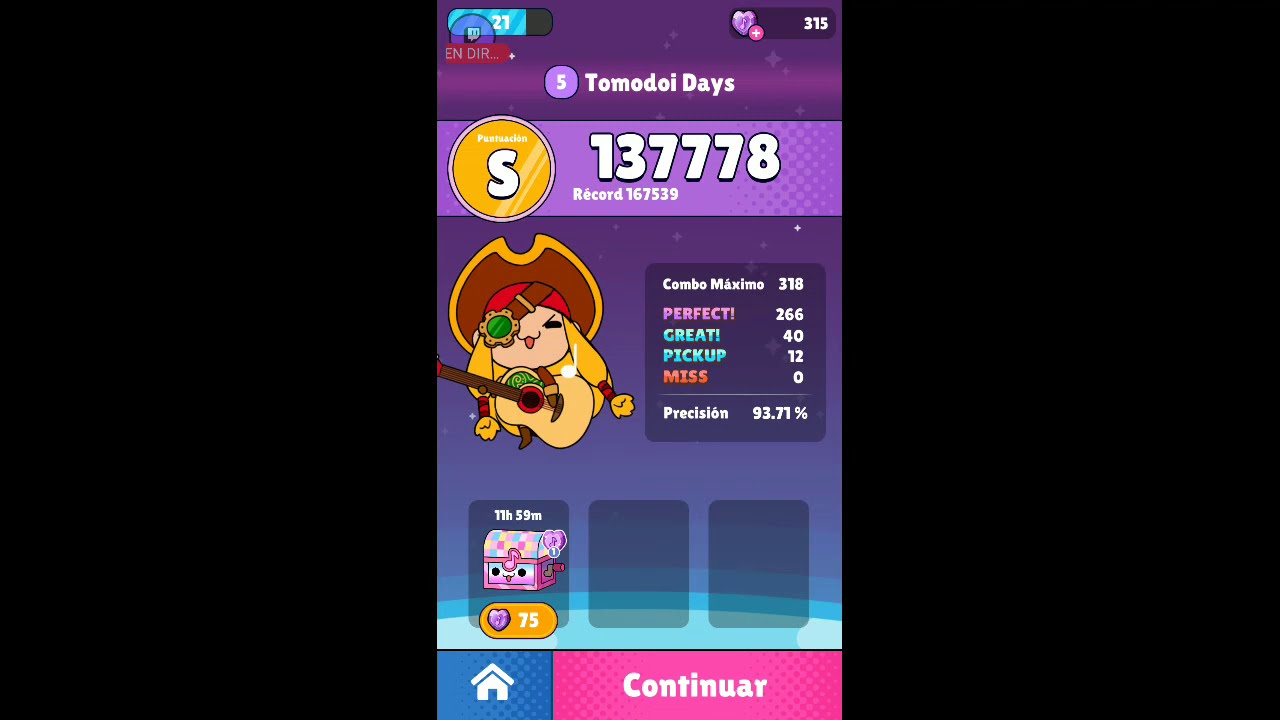This screenshot captures a vibrant mobile game interface, likely a rhythm game in Spanish, set against a gradient purple-to-aqua background. Dominating the left side is a cartoony female character dressed in a brown cowboy/pirate hat, a green eyepatch, and sporting green ponytails tied with red ribbons. She holds an acoustic guitar and is shown mid-performance. Adjacent to her, game stats are prominently displayed in a dark box: "Combo Máximo: 318," "Perfect: 266," "Great: 40," "Pickup: 12," "Miss: 0," and "Precision: 93.71%."

The top of the image features a light purple bar with large white text reading "Tomodoy Days 137,778" and below it, "Record 167,539." To the left of these stats is a yellow circle with a white "S" in the center. 

At the bottom of the screen, there are three dark boxes, with only the left one containing an image of a pastel-colored treasure chest that indicates "75 hearts" and a time of "11 hours 59 minutes." Further below, a yellow oval with a purple heart and "75" is visible. On the bottom left corner, a blue box with a white house icon is displayed, suggesting navigation to the home screen. Next to it, a pink button reading "CONTINUAR" in white letters offers a prompt to proceed. The scene is visually dynamic, with its mix of vivid colors, engaging character design, and detailed gameplay statistics.